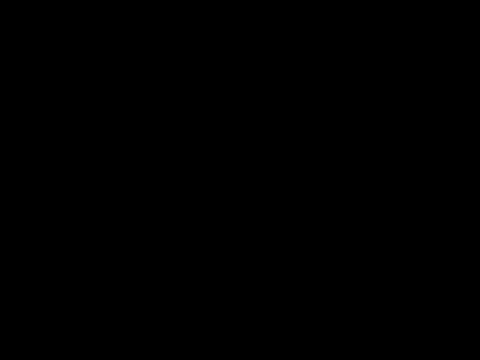This image is a rectangular plain black box, characterized by an infinite void of black darkness. The black background and black border present a jet-black screen with no discernible characteristics. There are no objects, people, animals, text, numbers, or any other elements visible. It is entirely devoid of any setting or style, embodying a vast expanse of dark nothingness.